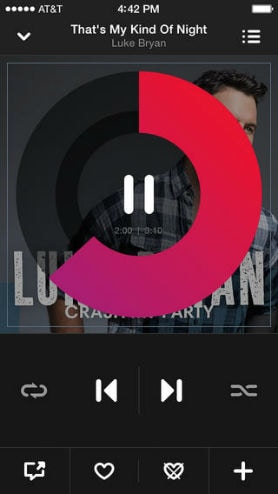This is a detailed screenshot of a video player interface displayed on a smartphone with AT&T service. The top of the screen shows signal strength with five dots on the left, the AT&T logo in the center, and the current time, 4:42 p.m., along with a full battery meter on the right. The central part of the screen features the song title "That's My Kind of Night" by Luke Bryan, set against a dark gray background. 

Adjacent to the song title on the right is a hamburger menu icon. Below the song title, there is a shot of the singer, who appears to be Caucasian, with short brown hair and wearing a plaid shirt. The name "Luke Bryan" is displayed over this image, along with some partially obscured text that appears to read "Crash the Party." 

A large circular playback icon overlays part of the singer’s image. This circular icon consists of a pause button in the center, surrounded by a translucent outer ring, a darker inner ring, and a partially filled solid red segment indicating the song's progress, which extends about two-thirds of the way around the circle starting from the 12 o'clock position. 

Below the circular icon, there are buttons for loop and crossfade functions, as well as backward and forward navigation. Further down, there is a horizontal array of interaction buttons: a speech bubble for comments, a heart icon, an X over a heart, and a plus button. These interaction buttons are separated by thin gray lines.